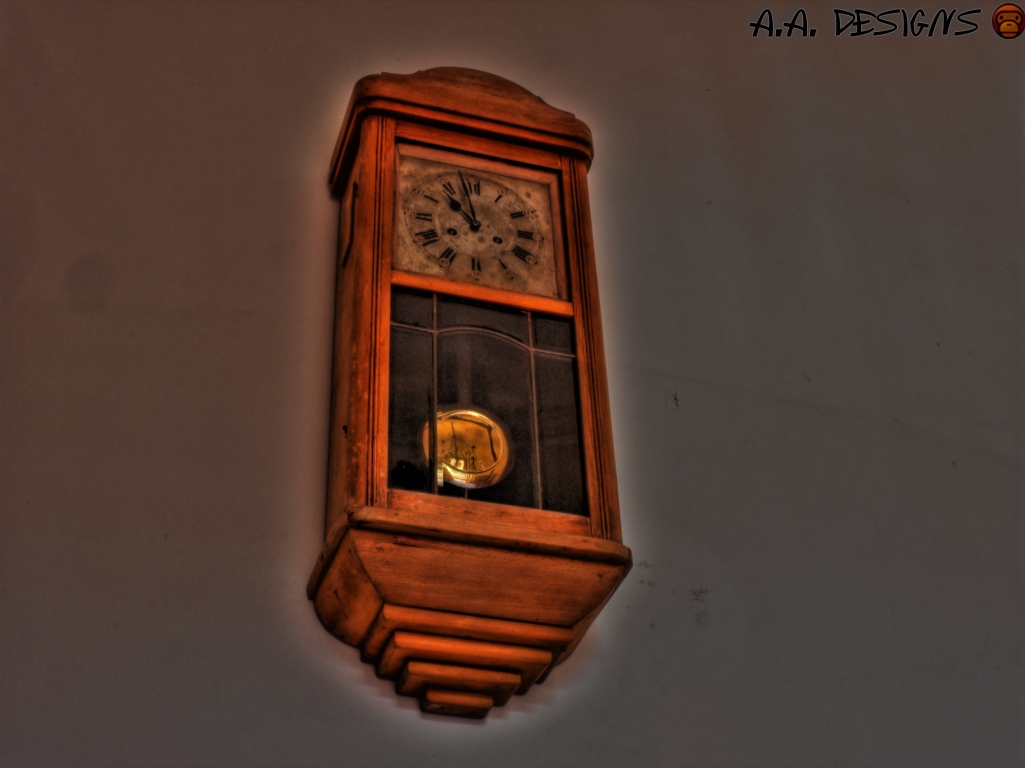The artwork features a classic, vintage-style wall clock prominently displayed on a gray-colored wall. Viewed from a bottom perspective, the clock boasts a beautifully crafted wooden frame and casing, enhancing its antique charm. Through the glass window of the wooden frame, a round, gold pendulum is visible, adding a touch of elegance to the piece. The clock face is adorned with Roman numerals, indicating that the time is nearly 11 o'clock. In the upper right corner of the image, the text "AA Designs" is inscribed, suggesting the creator of this intricate artwork.